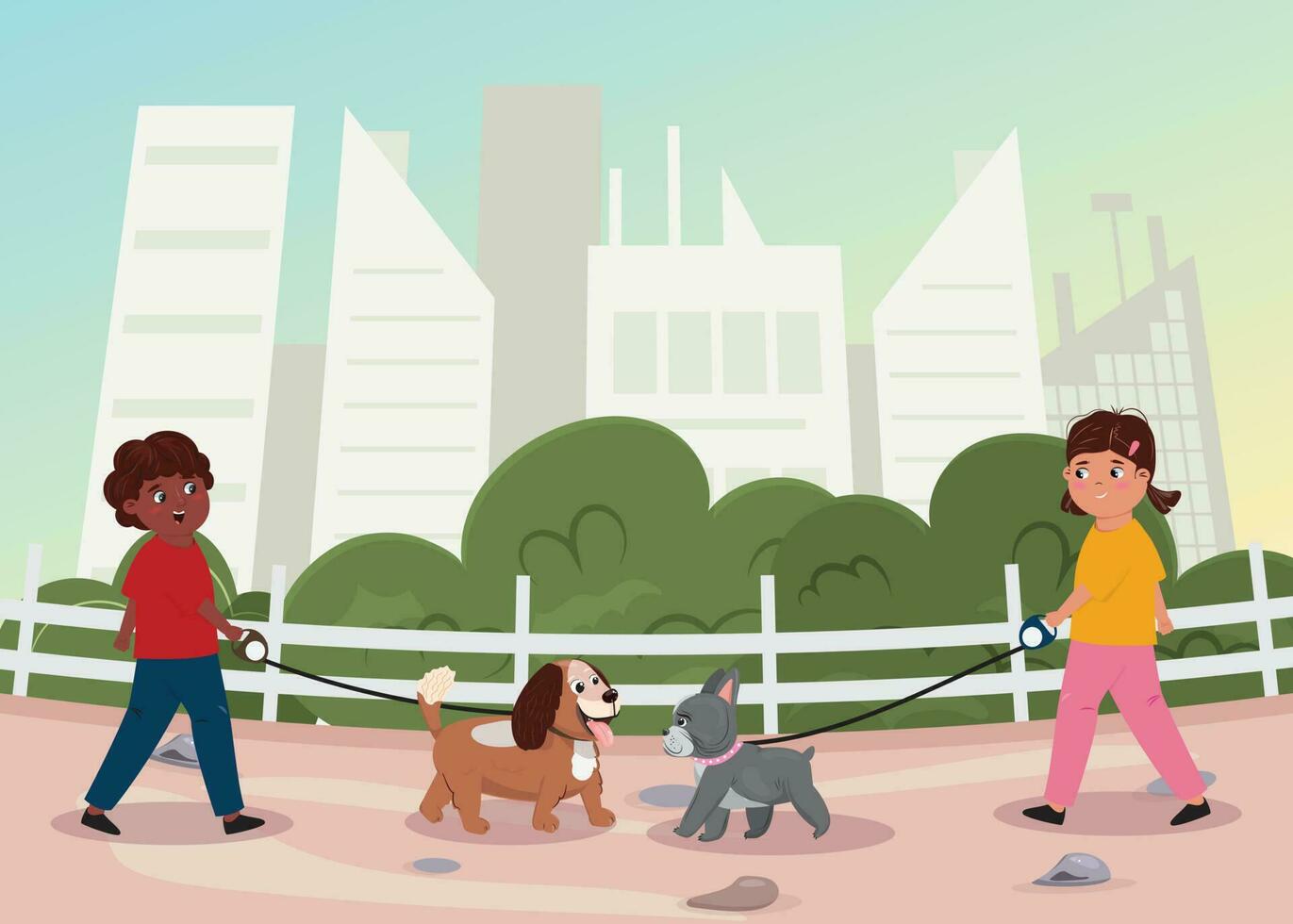The image is a vibrant, computer-generated cartoon illustration of two children walking their dogs, on a pink trail dotted with rocks, in an outdoor setting with a white picket fence, green bushes, and tall skyscrapers in the background against a greenish-blue sky. On the right is a Caucasian girl with brown hair styled in pigtails. She is wearing a gold short-sleeved top, pink long pants, and black shoes. She holds a black retractable leash attached to a gray, short-haired dog with a pink collar and a white muzzle. On the left is an African American boy with curly brown hair, dressed in a red short-sleeved t-shirt, blue pants, and dark shoes. He holds a retractable leash connected to a brown and white dog with long ears, its tongue hanging out. The two kids, both around 10 to 12 years old, walk towards each other as their dogs, about to greet and sniff each other, add a delightful moment to the scene.